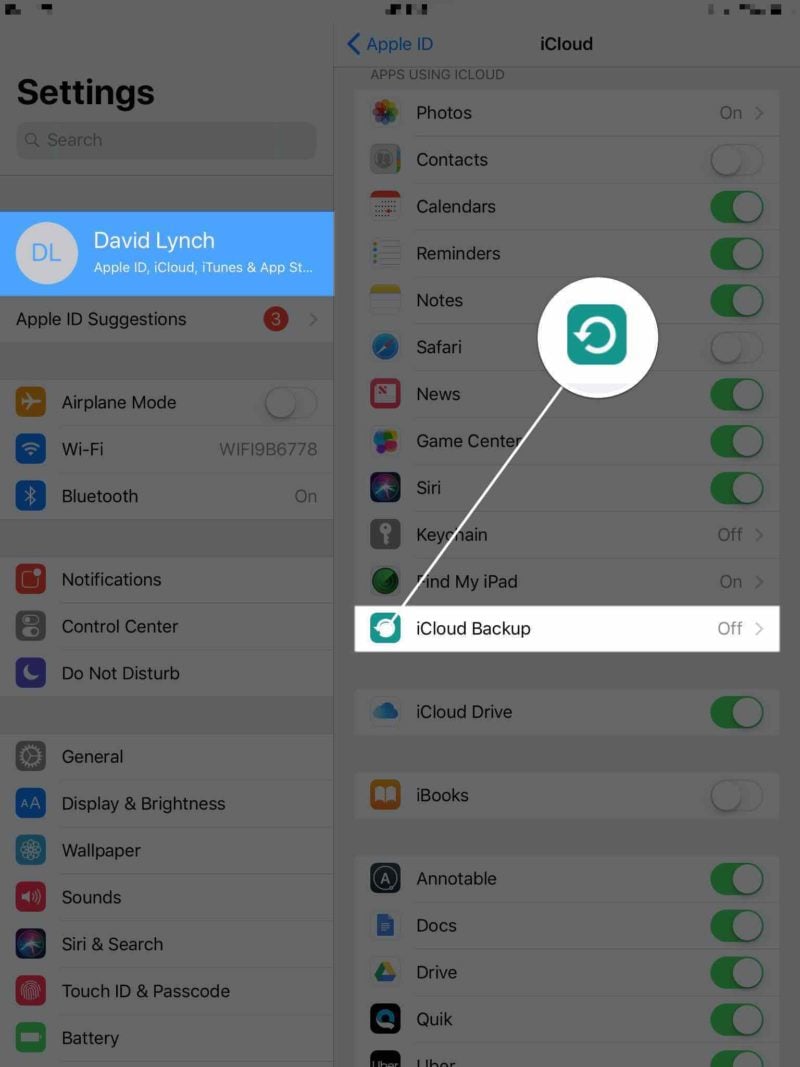This image captures the settings page of an iPhone, focused on the Apple ID section. At the top of the screen, the word "Settings" is prominently displayed, though the overall image appears greyed out except for specific highlighted areas. The username "David Lynch" is prominently featured in bold light blue text, accompanied by the initials "DL" inside a circle to the right of the name. Directly below, the options for "Apple ID, iCloud, iTunes & App Store" are visible. This section has been expanded to reveal various linked services and settings. Among them, the "iCloud Backup" feature stands out, connected by a line to its corresponding circular arrow symbol, indicating recent activity or a highlight. The detailed layout offers a clear view of the different settings and options associated with the Apple ID.